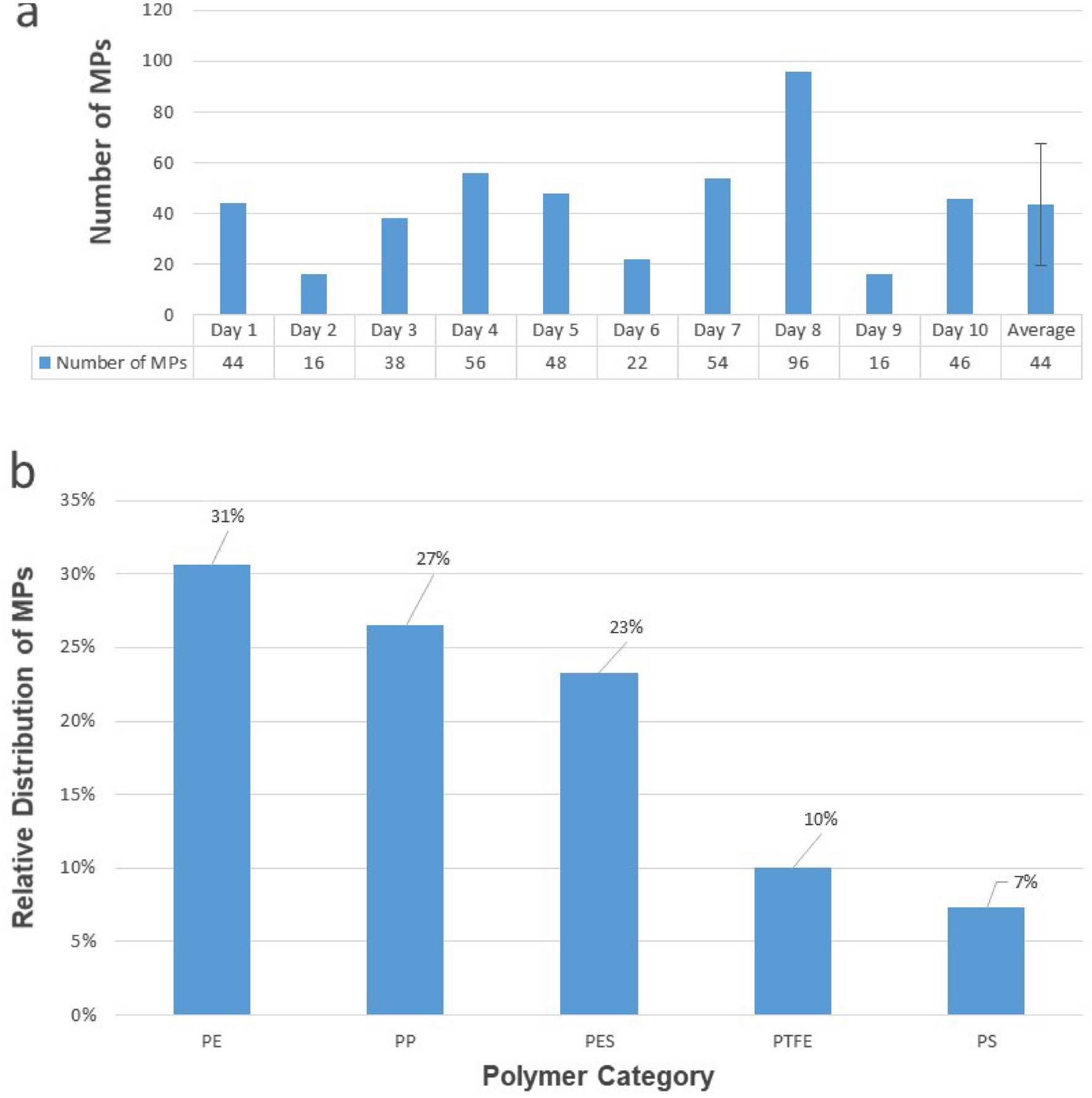The image contains two bar graphs on a white background, likely designed for slideshows or handouts, focusing on the number and distribution of MPs. The first bar graph (Graph A) presents the number of MPs recorded over ten days, plus an average. Specifically, Day 1: 44 MPs, Day 2: 16 MPs, Day 3: 38 MPs, Day 4: 56 MPs, Day 5: 48 MPs, Day 6: 22 MPs, Day 7: 54 MPs, Day 8: 96 MPs, Day 9: 16 MPs, Day 10: 46 MPs, with an average of 44 MPs. The vertical axis measures the number of MPs, labeled accordingly from bottom to top. The second bar graph (Graph B) illustrates the relative distribution of MPs across various polymer categories, ranging from 0 to 35% on the vertical axis. The polymer categories are listed at the bottom in black text, being PE (31%), PP (27%), PES (23%), PTFE (10%), and PS (7%). Both graphs utilize blue bars with black text for clear data visualization.